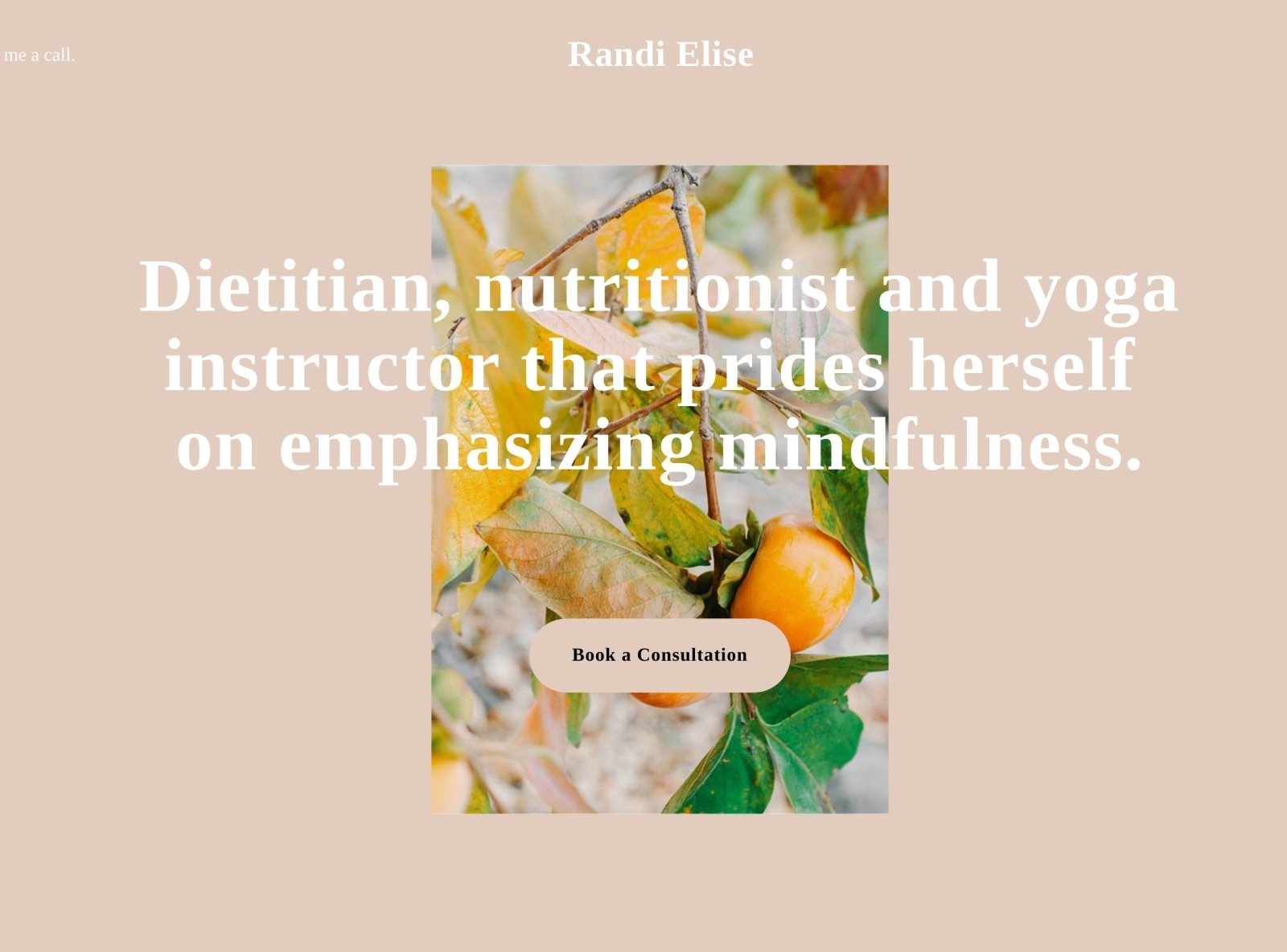The image features a cream-colored rectangular background. At the top center, in prominent white text, is the name "Randy Elise," with both 'R' and 'E' capitalized. Directly below the name is a picture depicting lush green leaves and a small fruit that resembles either a berry or an apple growing from a plant. Below the image, there is a cream-colored button, matching the main background shade, adorned with black text that reads "Book a Consultation."

Above the button, in a larger white font, the following description is displayed: "Dietician, Nutritionist, and Yoga Instructor that prides herself on emphasizing mindfulness." This structured layout suggests that the image is part of a health and wellness website where users can connect with Randy Elise, a professional who specializes in dietary guidance, nutrition, and yoga for enhancing well-being. By clicking the centrally positioned button, users can book a consultation with her.